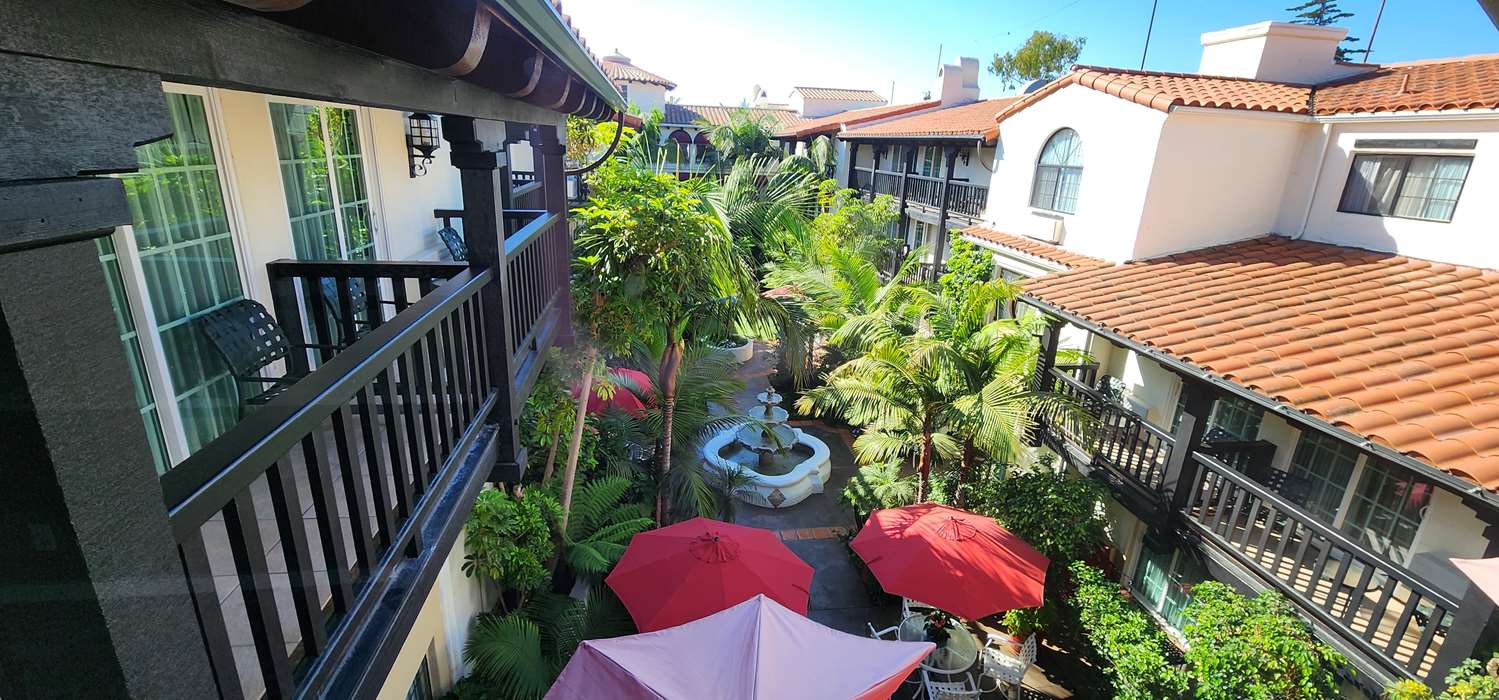This image appears to be taken from a second or third-story balcony, offering an overlook into a picturesque Spanish-style courtyard. Centered in the courtyard is a three-tiered fountain, with the largest basin at the bottom, a medium basin in the middle, and the smallest at the top, all holding glistening water. Surrounding the fountain are several patio tables equipped with vibrant umbrellas, including red and pink ones, providing shade and color to the scene. The courtyard is lush with trees that resemble palm trees, adding a tropical feel. The building to the right features a brown, terracotta roof typical of Spanish architecture, with a black-railed balcony and several windows. Similarly, the left side showcases another balcony with a black railing, framed by a bright blue sky and more trees in the background, suggesting a sense of openness and tranquility. This overall setting feels like it could be part of a resort or apartment complex designed in a Mediterranean style.